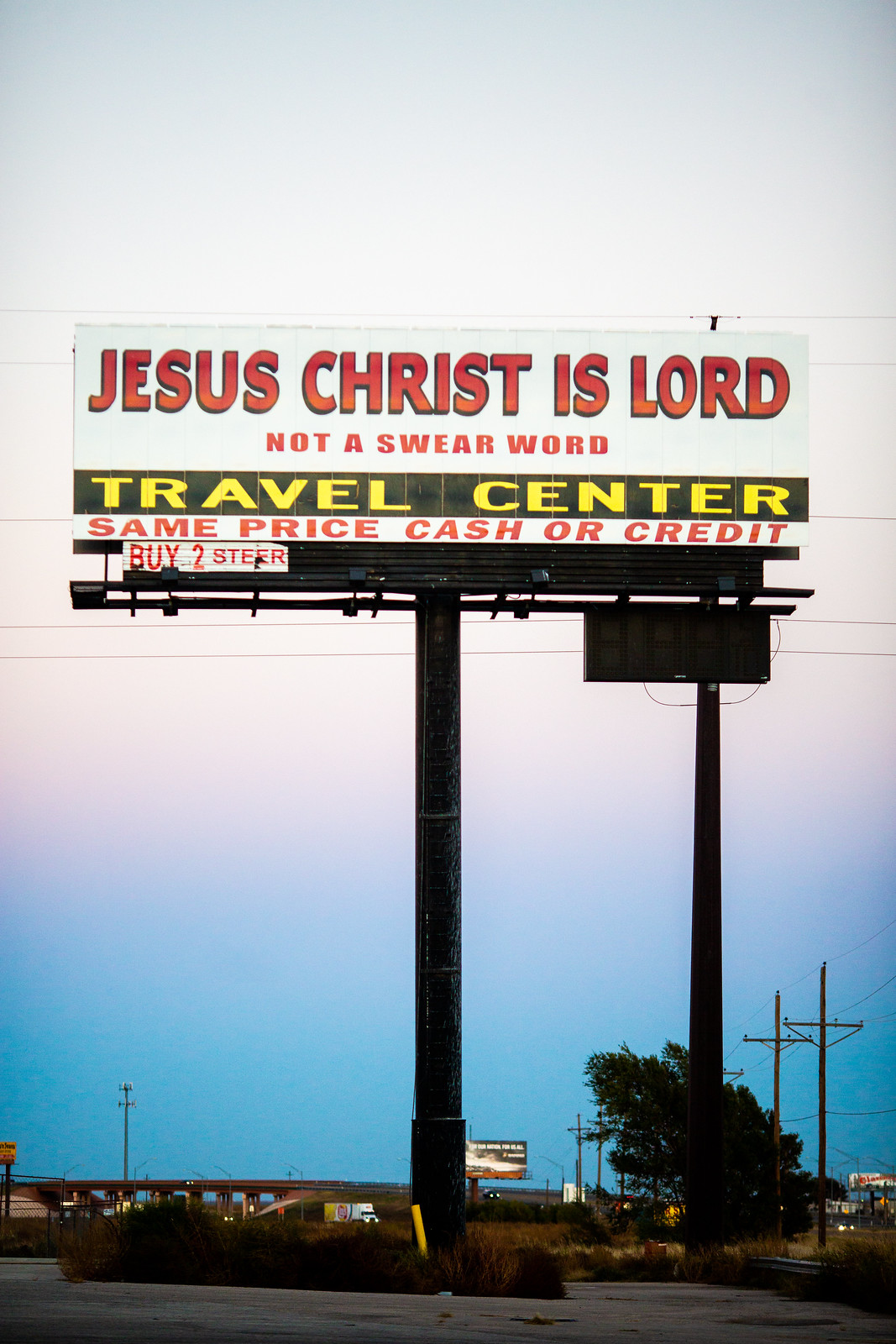This image captures a duo of towering billboards, silhouetted against a striking sky that transitions from deep blue at the horizon to bright white towards the top, suggesting that the sun is setting. In the background, the details are obscured, but to the right of the billboards, power poles are visible. A prominent feature is the large cell phone tower and a substantial bridge in the distance. On one of the billboards, large red letters proclaim, "Jesus Christ is Lord, not a swear word." Below this, the billboard advertises a Travel Center with a statement, "same price, cash or credit," and a promotional message, "buy two steer." A leafy tree or bush partially obstructs the view of one of the signs, adding a touch of nature to the otherwise industrial scene.